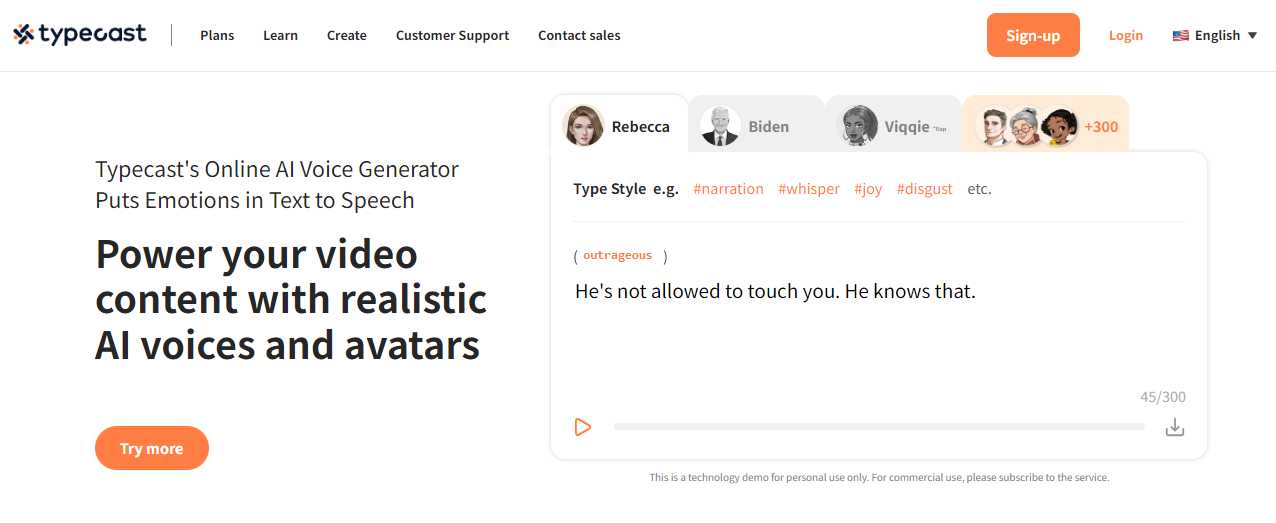This is a screenshot taken from a website called "Typecast". At the top of the image, there is a prominent header displaying the word "Typecast" in black print, accompanied by a unique tic-tac-toe board emblem placed sideways on either side of the word. To the right of the "Typecast" logo, there is a navigation bar with several smaller print options: "Plans," "Learn," "Create," "Customer Support," and "Contact Sales". 

On the same top line, there is a blank space followed by a bright orange "Sign-Up" button positioned towards the right. The button stands out with "Sign-Up" written in white, easy-to-read text. Next to the "Sign-Up" button, there is a "Login" section, and further to the right, there is a drop-down menu that says "English" accompanied by an American flag, indicating language options for the site.

As you move down the page, on the left-hand side, there is a slogan in bold lettering: "Typecast online AI voice generator puts emotions in text to speech." Below this, there is another sentence: "Power your video content with realistic AI voices and avatars." Beneath this promotional text, an orange button labeled "Try More" invites users to explore further.

On the right side of this section, there are names listed—Rebecca, Biden, Viggie—followed by the phrase "plus 300 more," indicating the variety of AI-generated voices available for users to try.